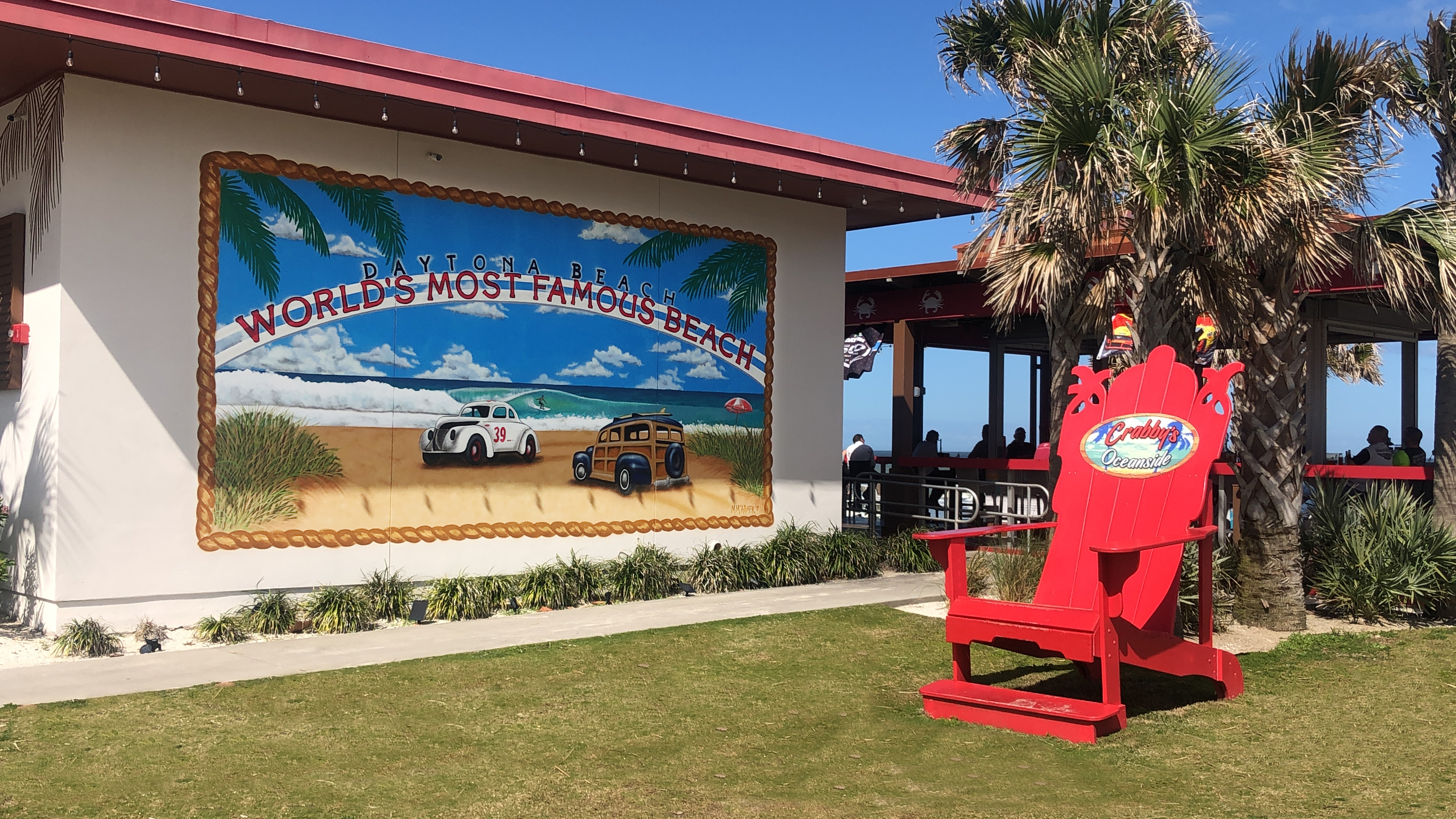This color photograph captures a vibrant scene in Daytona Beach, highlighting both natural and man-made features. Dominating the foreground is an oversized red lifeguard chair emblazoned with "Krabby's Oceanside" in red and white text, suggesting it serves as a whimsical photo spot for tourists. The chair is surrounded by lush, freshly cut green grass and stands in front of a grouping of palm trees, one prominently featured on the right and another partially visible. To the left of the chair is a beige building adorned with a mural that proclaims "Daytona Beach, World's Most Famous Beach" in bold black and red lettering. The mural vividly depicts a sandy beach with waves, alongside classic vehicles, including a white car with the number 39 in red and a brown car trimmed in black, evoking a nostalgic coastal vibe. The building is topped with a red roof and draped with hanging lights, adding a festive atmosphere. Adjacent to it, people can be seen sitting in what appears to be a picnic area, enjoying the sunny, blue-skied day while gazing towards the pier and the ocean. The scene seamlessly blends tropical charm with cultural landmarks, encapsulating the spirit of Daytona Beach.